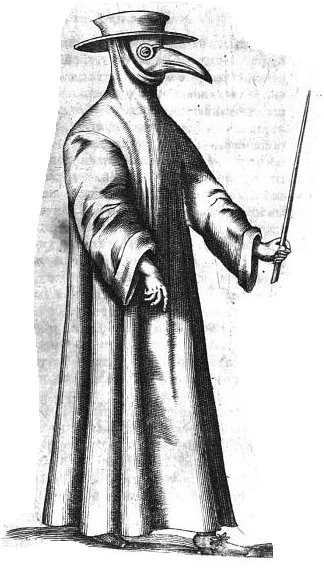This black and white image appears to be an illustration that resembles historical artwork from a book, magazine, or newspaper. It depicts a figure dressed like a doctor from the time of the Black Plague. The doctor is wearing a long, baggy robe and a distinctive hat. A notable feature is the elongated, beak-shaped mask covering his face, which resembles a bird's beak and is complemented by round glasses. In his left hand, he holds a long stick or cane, while his other hand points downward. He is also depicted with flat shoes on his feet, walking. The entire scene is in black and white, capturing the eerie and unsettling appearance of the historical plague doctor.